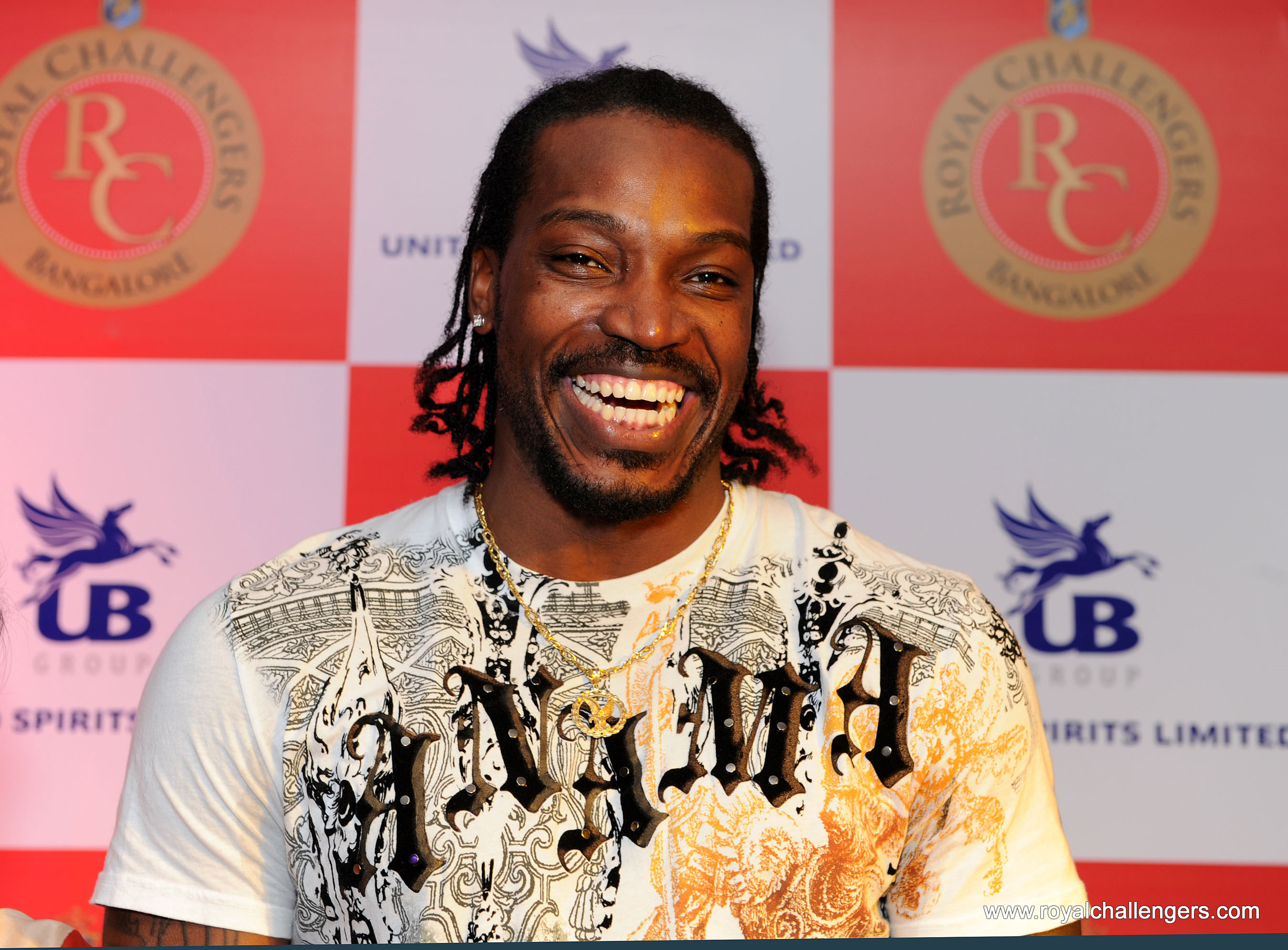The image features cricketer Chris Gayle at what appears to be a press event. He is smiling and looking directly at the camera, showcasing his large, beaded, braided long hair, a subtle mustache, and a small beard. Chris is wearing a white t-shirt adorned with various black, yellow, and orange designs and the word "NAMA" in a decorative font. Around his neck, he sports a gold chain with a circular pendant and he also has an earring on his right ear. The background features a red and white checked banner displaying both the Royal Challengers Bangalore IPL team logo and the United Spirits Limited logo with the tagline "Spirits Unlimited." At the bottom right corner of the image, the source "www.royalchallengers.com" is visible.